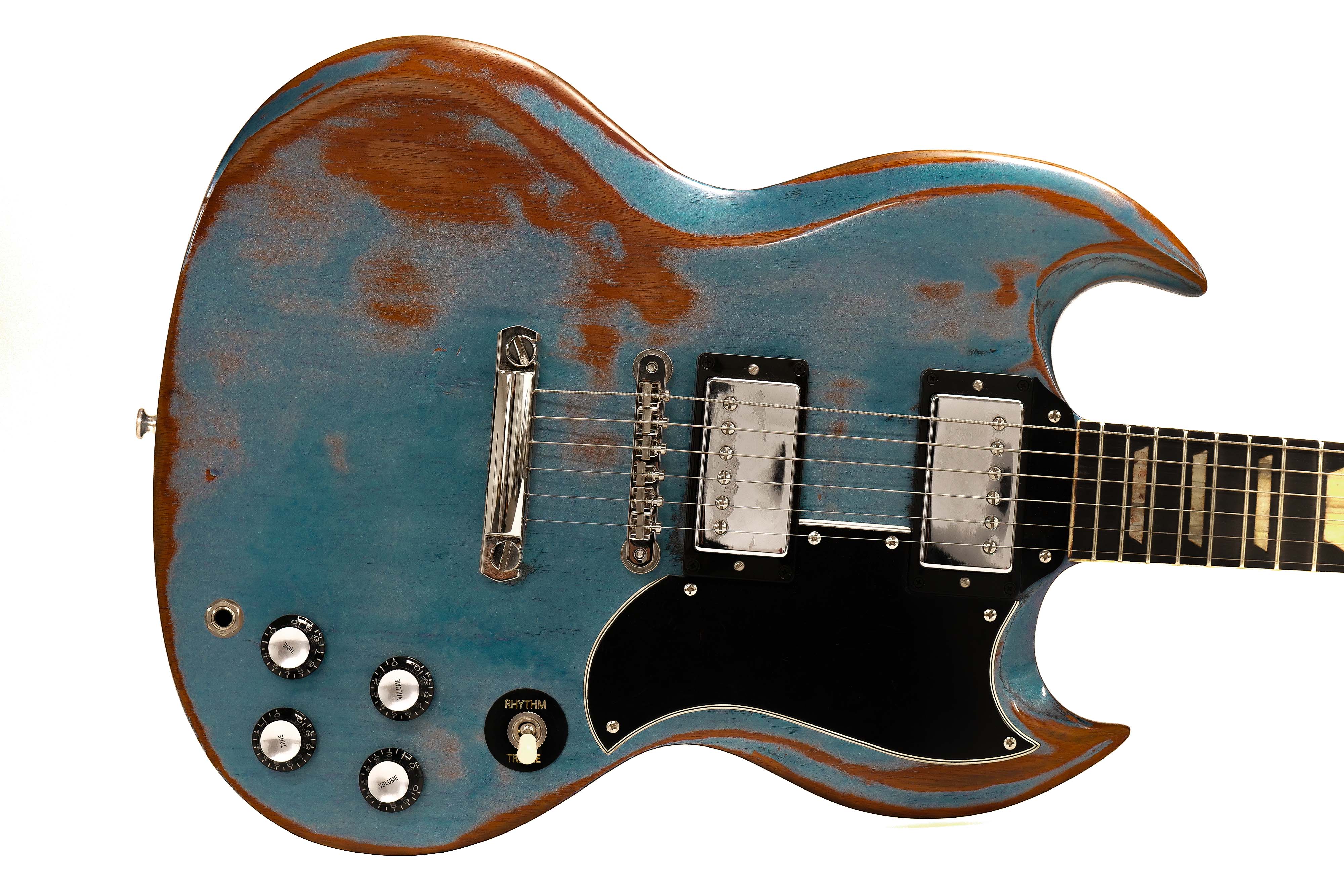This photograph captures a vintage guitar, reminiscent of the 1950s era, exuding both charm and character. The body of the guitar is prominently featured and fades into a partial view of the neck. Painted in a light blue hue, the guitar’s surface displays natural wear, with peeling paint and spots where an orangish rust color has emerged. At the bottom, there is a notable silver circular piece, possibly a decorative element, also showing signs of peeling. Positioned on the body is a silver switch encircled by a black ring, adding to its functional yet antique aesthetic. Chrome detailing is evident around the string area, complemented by black accents, enhancing its vintage appeal. A black section with silver rivets further accentuates the guitar's classic design. The overall visual speaks to a bygone era, making this guitar a captivating piece for any vintage enthusiast.